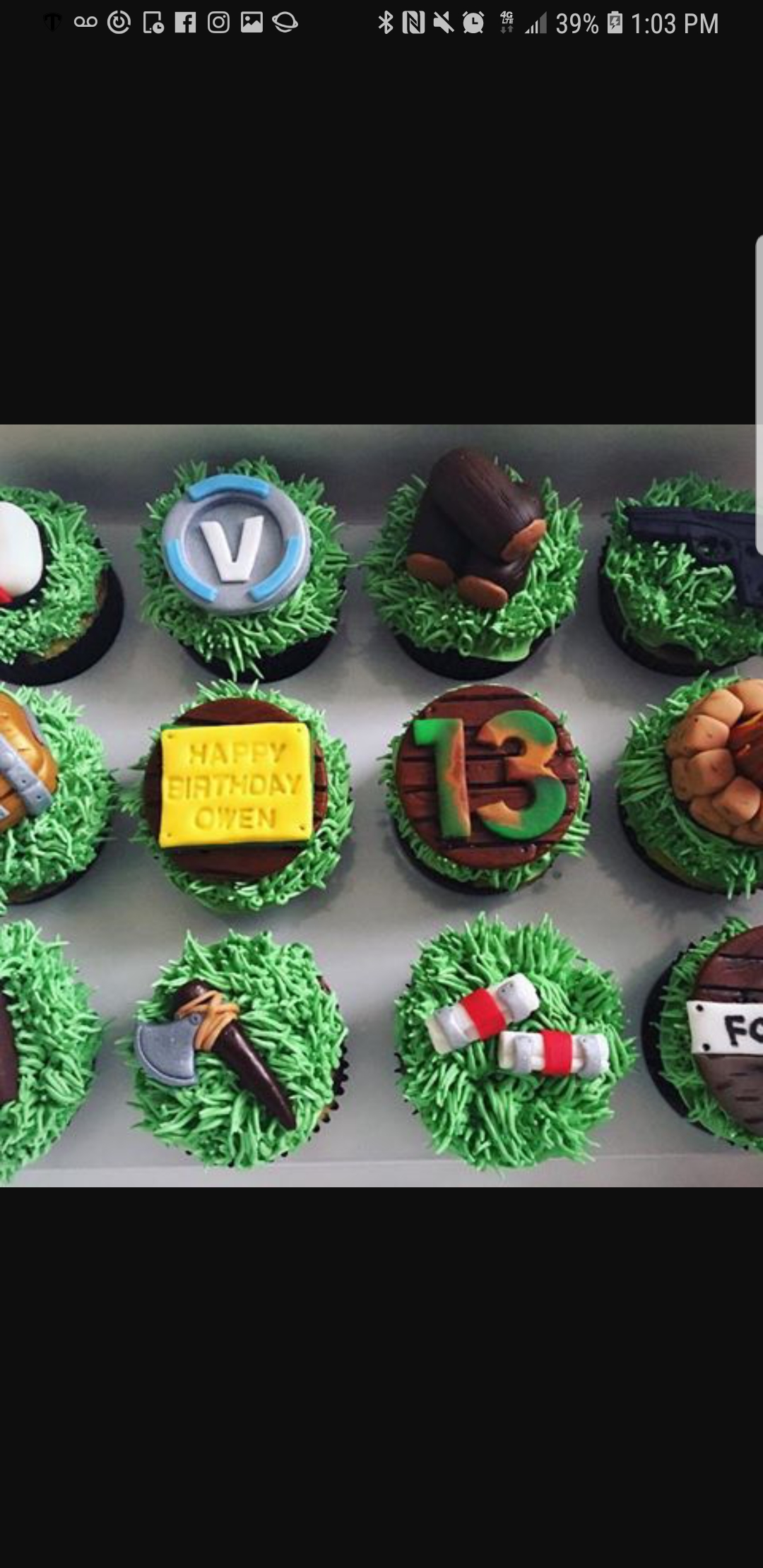This image appears to be a screenshot taken from a cell phone, showing a dozen elaborately decorated cupcakes arranged on a white tabletop, with the top and bottom of the image featuring black bars where the phone's display ends. The cupcakes, likely for a birthday celebration, are adorned with a unified green grass-like frosting. 

Distinct decorations embellish each cupcake: 

1. A white medallion with a "V" on it.
2. Three stacked chocolate logs.
3. A half-visible object, likely an element of the theme.
4. A yellow plaque reading "Happy Birthday Owen".
5. The number "13" in green and orange.
6. A half-visible cupcake, partially cut off from the screenshot.
7. Another half-visible cupcake.
8. A small hatchet or axe.
9. Two white items with red bands, possibly resembling packages or weights.
10. Another half-visible cupcake.
11. A nearly obscured sign with an "F".
12. A black shape resembling a gun.

The design of these cupcakes suggests a possible lumberjack or an outdoor adventure theme, reinforced by elements like the axe, logs, and the green grass frosting. Despite some ambiguity in a few decorations, the detailed elements contribute a cohesive and meticulously thought-out visual aesthetic.